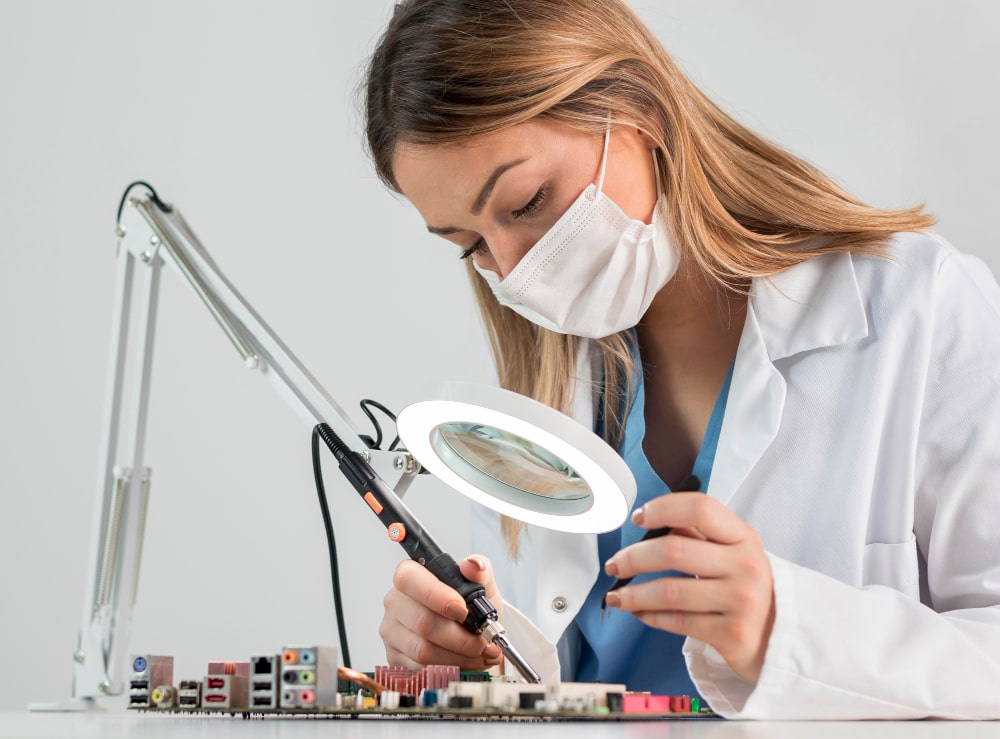In the image, a sandy blonde-haired woman with shoulder-length hair is seated at a desk, focused intently on her work with an electrolyte panel. She is fully attired in a professional ensemble that includes a white lab coat worn over a light blue nurse uniform with a V-shaped collar, and a white surgical mask covers her face. She is holding a black tool with a silver tip—likely a soldering iron, positioning it meticulously on the circuitry of the electrolyte panel beneath her. Her gaze is directed through a large circular magnifying glass mounted on a white arm, which in turn is attached to a silver support positioned to the left side of the image. This setup is staged against a pristine white background, suggesting the image may be a stock photo, meticulously crafted to represent a STEM environment, particularly highlighting women's involvement in scientific and technical fields. Every detail, from her neatly maintained eyebrows to the well-organized work setting, enhances the impression of a clean, perfect, almost too ideal environment.